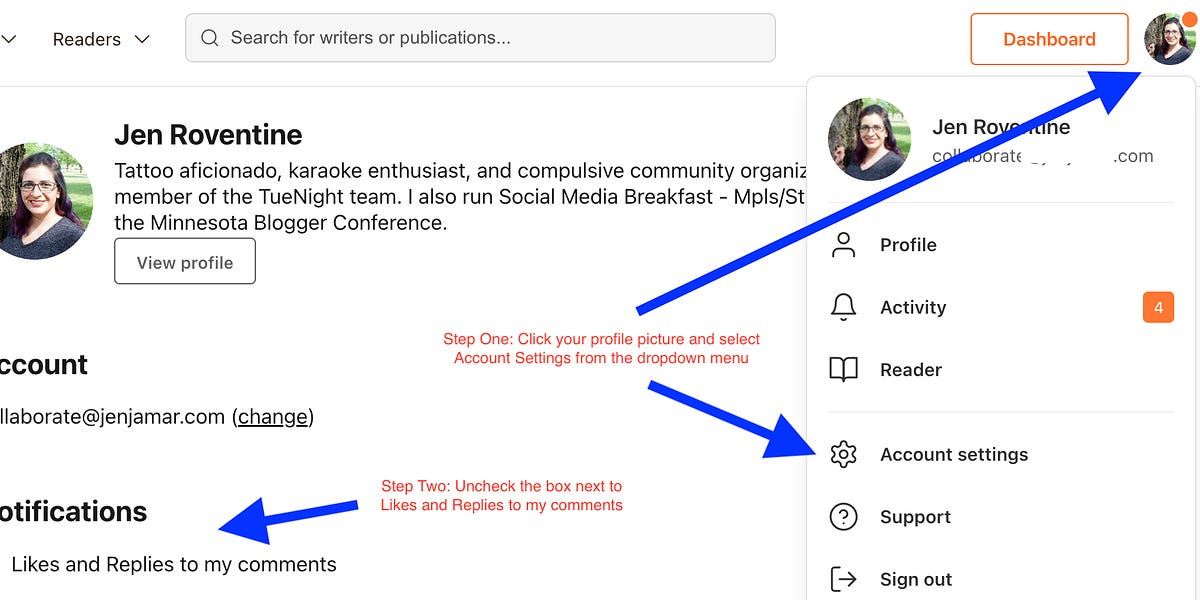The image shows a detailed view of a website interface, specifically the home page of a user named Jen Roventine. At the top right corner of the page is Jen's profile photo, accompanied by a dashboard button. Clicking on her photo reveals a drop-down menu with the following options: Profile, Activity, Reader, Account Settings, Support, and Sign Out.

The main section of Jen's home page showcases her profile information, which reads: "Jen Roventine, tattoo aficionado, karaoke enthusiast, and compulsive community organizer. Member of the Tune Night team. I also run Social Media Breakfast and the Minnesota Blogger Conference."

Below this information, there is a "View Profile" button.

Overlaying Jen's profile photo are annotated blue arrows and steps providing instructions. The steps are as follows:
1. Click the profile picture and select "Account Settings" from the drop-down menu.
2. Uncheck the box next to "Likes and Replies to My Comments" to stop receiving notifications. Additionally, there is a note indicating that you can change your email address under the Account section.

These annotations and steps are designed to guide users through adjusting their notification and account settings.